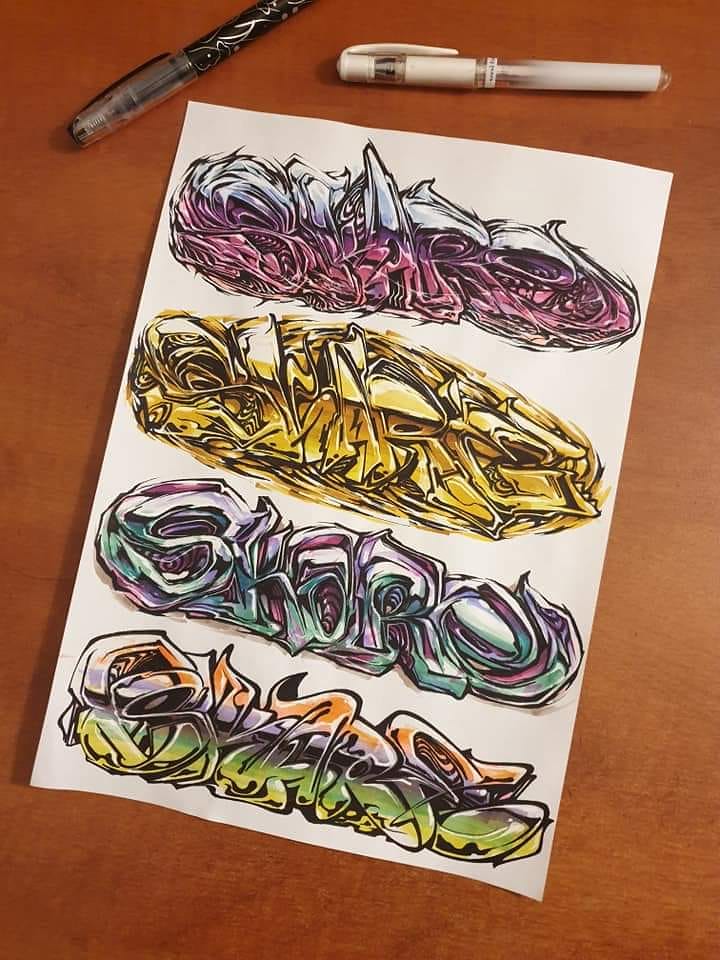The image showcases a detailed drawing on a white piece of paper, which is placed on a medium-shaded wooden surface. The artwork features four distinct graffiti-style tag designs, each characterized by vibrant colors and bold, black outlines. The first tag incorporates a mix of pink, purple, and off-silver white, outlined in black. The second tag showcases various shades of yellow also highlighted with black outlines. The third design combines purple, off-silver white, and teal greenish blue hues. The fourth tag blends orange, white, purple, silver, green, and yellow elements. Above the paper, two pens are visible: one is black with silver swirls on the body and a clear cap, while the other is white with a white cap and a semi-transparent body.